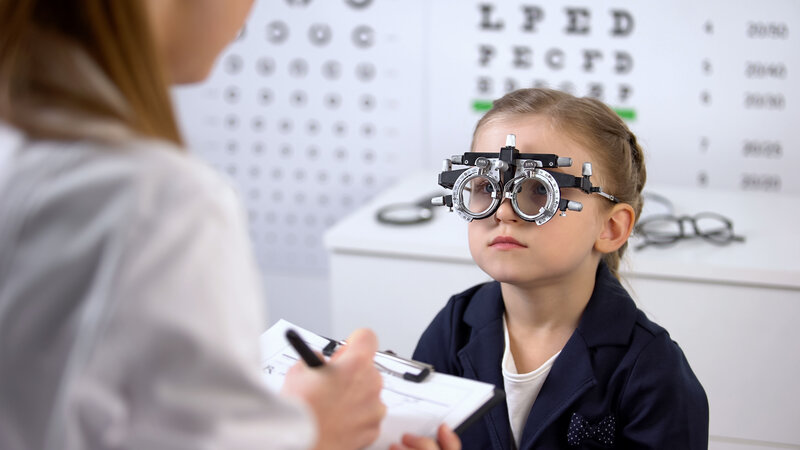In the optometrist's office, a little girl with light brown hair braided back is seated on a stool in front of a white counter. She is wearing a blue blazer over a white t-shirt and has a piece of optometric equipment over her eyes, used to determine her prescription. In the background, an entire wall is adorned with various eye charts, and several pairs of eyeglasses are scattered on the counter. Facing the girl is a female optometrist, identifiable by her long hair and white lab coat. Though her face is mostly out of focus, it is clear she is holding a clipboard with papers and writing with a black pen. The scene captures a moment of eye examination with the clinical ambiance indicated by the eye charts and the array of eyeglasses.